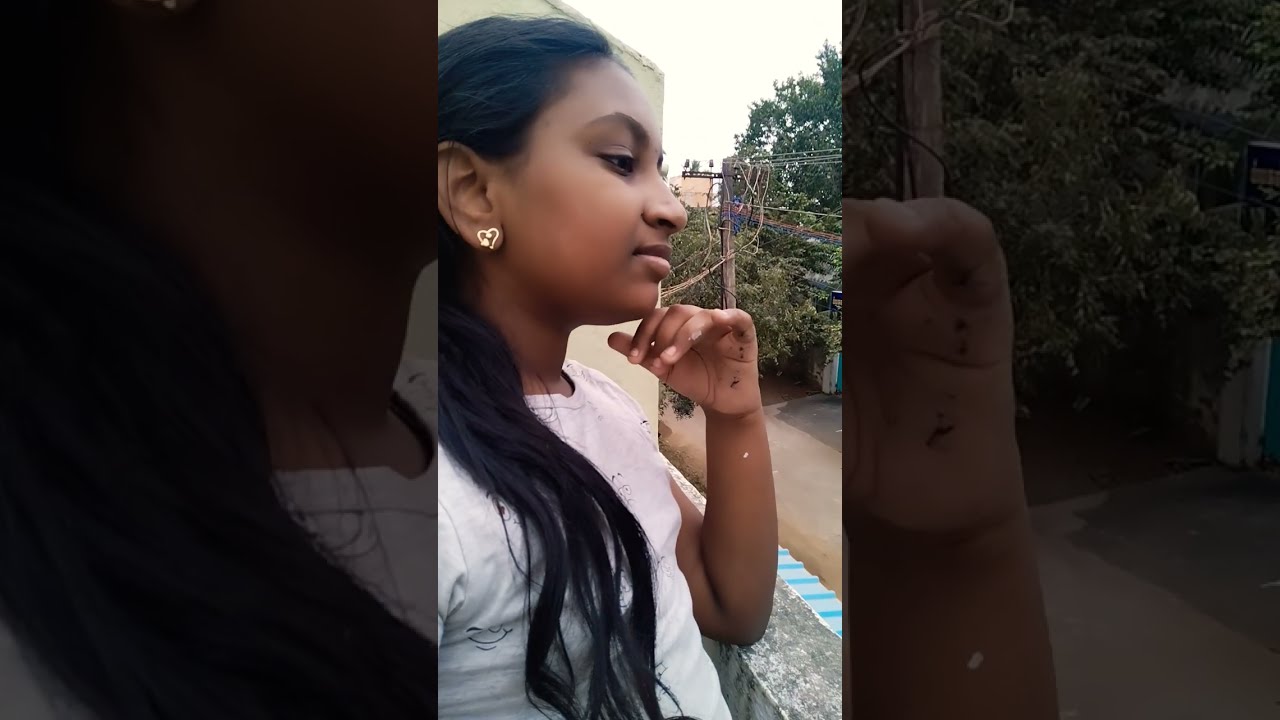The image shows a young teenage girl, likely around 13 or 14 years old, with dark skin and very long black hair draped over her shoulder. She wears a white short-sleeved top and a small gold heart earring. The girl appears to be lost in thought, looking out into the distance with a melancholic expression while leaning on a gray cement balcony with her left elbow. Her hand is near her chin, and there is an indistinct marking on it, possibly a tattoo, dirt, or a wound. The background reveals a dirt road with black cement patches, green trees, and some telephone poles with wires. The sky is mostly gray, casting a bright glare. Below the balcony, a blue and white awning is visible. The sides of the image are darkened and feature enlarged, grayed-out portions of the main image to frame the scene without distraction. The setting suggests it might be in another country, adding a sense of mystery and cultural context to the photograph.